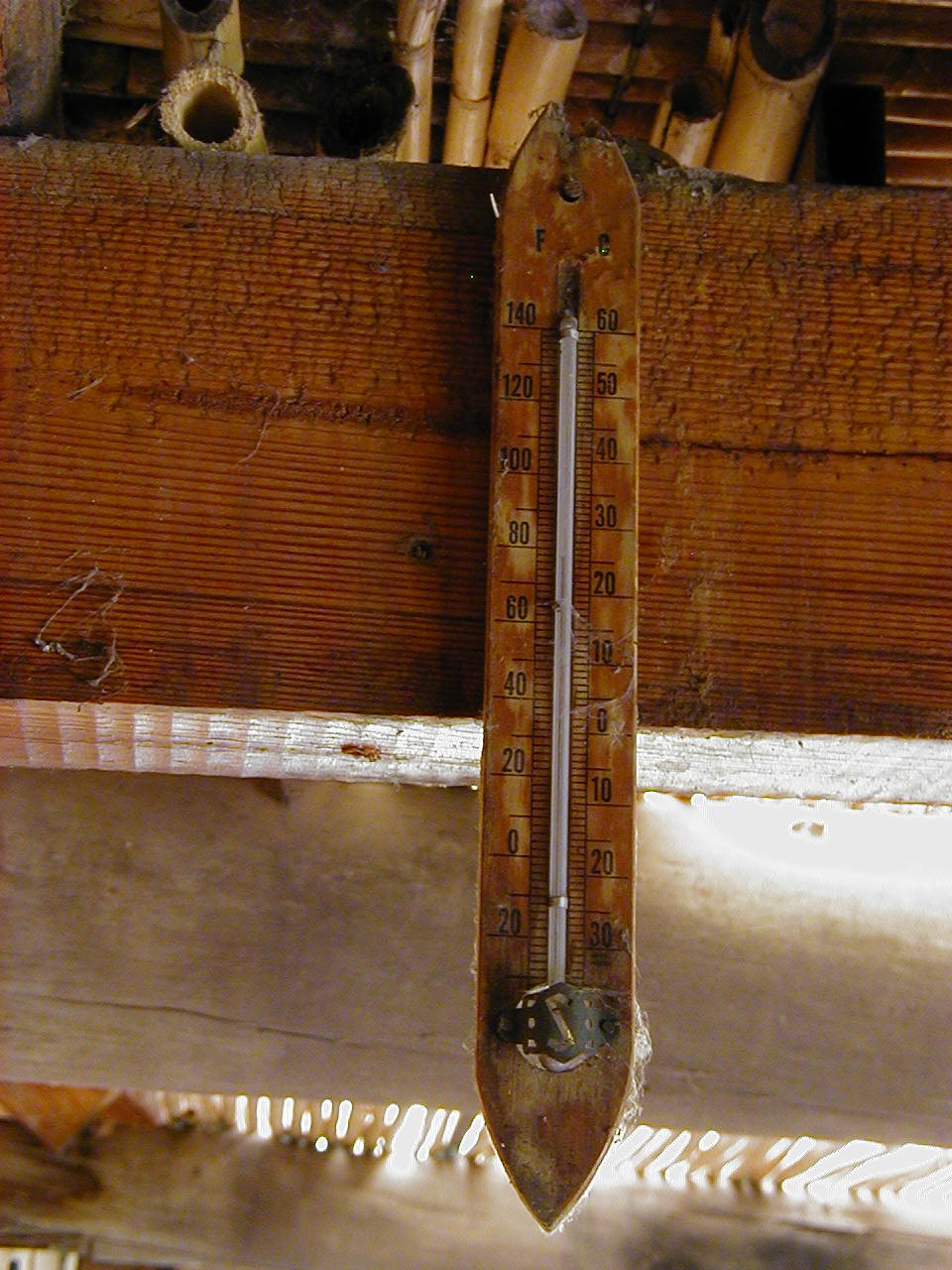A vertical mercury thermometer, primarily made of wood, features a thin, rectangular body with a pointed bottom. The thermometer displays Fahrenheit temperatures on the right side, ranging from -20 to 140 degrees, and Celsius temperatures on the left side, ranging from -30 to 60 degrees. The current reading indicates approximately -11 degrees Fahrenheit. This thermometer is mounted on a wooden board, possibly part of a ceiling or bookcase, as suggested by the bamboo tubes positioned above it. The board shares a similar light brown hue to the back of the thermometer, while the shelf itself is a darker wood. The setting appears to be inside a wood cabin, with light filtering through a skylight adorned with bamboo slats, providing a rustic and warm ambiance.